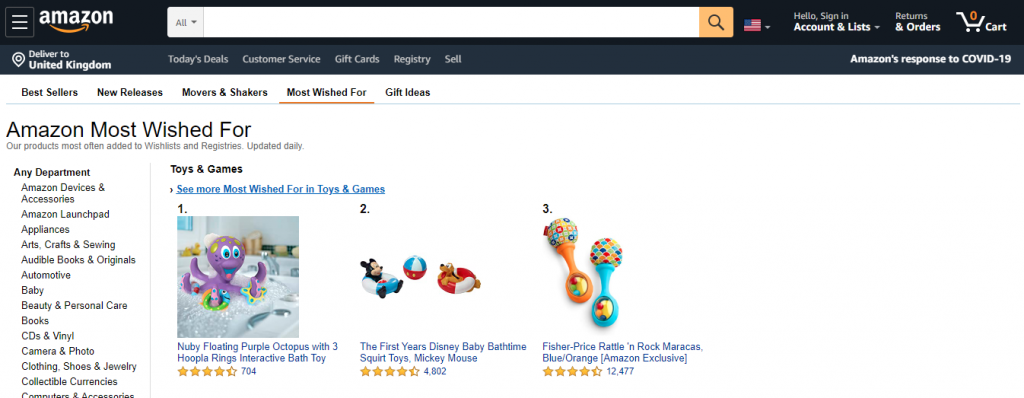On the Amazon Toys and Games page, the screen displays familiar Amazon interface elements. At the top left, there is a three-line menu icon, followed by the Amazon logo, which is white text with a yellow smile and a right-pointing arrow below the "Z". Adjacent to this, a gray box labeled "All" offers a drop-down menu to select different categories. A white search bar is next to this, along with a yellow search button featuring a magnifying glass icon. 

To the right, an American flag icon with a drop-down menu allows the selection of different languages. There is also a "Hello, Sign in" link, an "Accounts & Lists" drop-down menu, and "Returns & Orders" option, both of which are clickable. The shopping cart icon shows a "0", indicating no items have been added to the cart yet. Below, a gray rectangular pin icon with the text "Deliver to United Kingdom" in white is visible.

Further down, a grayscale menu presents options like "Today's Deals", "Customer Service", "Gift Cards", "Registry", and "Sell". To the right, there is a white text link titled "Amazon's response to COVID". 

Beneath this, another menu features "Bestsellers", "New Releases", "Movers and Shakers", "Most Wished For", and "Gift Ideas" on a white background. "Most Wished For" is highlighted with an orange underline and the text "Amazon's Most Wished For: Our products most often added to wish lists and registries, updated daily" appearing below. 

On the left side, an expanded menu titled "Any Department" lists categories like "Amazon Devices & Accessories", "Amazon Launchpad", "Appliances", "Arts, Crafts & Sewing", "Audible Books & Originals", "Automotive", "Baby", "Beauty & Personal Care", "Books", "CDs & Vinyl", "Camera & Photo", "Clothing, Shoes & Jewelry", "Collectible Currencies", and "Computers & Accessories" before being cut off. A faint gray bar separates this menu from the main page.

In the main section, there are headings "Toys and Games" and "Most Wished For in Toys and Games" as clickable blue links. 

Highlighted items include:
1. **Newbie Floating Purple Octopus with Three Hoop Rings Interactive Bath Toy** (image of an octopus in a bathtub with rings). It has a rating of 4.5 stars from 704 reviews.
2. **The First Years Disney Babies Bath Time Squirt Toys Mickey Mouse** (image of Mickey Mouse and Goofy in an inner tube with a beach ball). It is rated 4.25 stars by 4,802 reviewers.
3. **Fisher-Price Rattle and Rock Maracas Blue and Orange Amazon Exclusive** (image of two multicolored rattles in blue and orange). It enjoys a 4.5-star rating from 12,477 reviews.